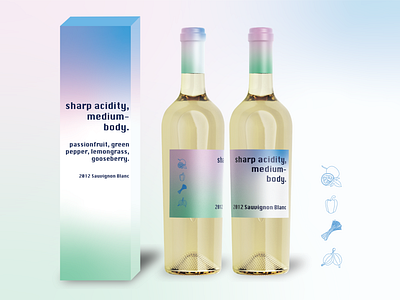A captivating advertisement features three items prominently displayed against a pristine white background: a tall, colorful liquor bottle box and two corresponding wine bottles. The box, standing on the left, flaunts a gradient design that transitions from teal green at the base, through white, to a serene pinkish-purple, finishing with sky blue at the top. Bold black text imprinted on the central white strip reads "sharp acidity, medium body," with additional descriptors such as passion fruit, green pepper, lemongrass, and gooseberry, though smaller text remains difficult to discern.

To the right of the box, two wine bottles, containing a light, pale tan liquid, mirror the box's pastel palette in their labels and foil wraps. The label colors echo the teal, white, and sky blue gradient, adding touches of pink, consistent across all items. The bottle on the right particularly highlights "sharp acidity, medium body" in prominent dark script, with faint illustrated icons hinting at the unique flavor profile. These Sauvignon Blanc wines, possibly from the 2021 vintage, are presented elegantly, making a visually striking and informative display centered on their distinct sharp acidity and medium body characteristics.